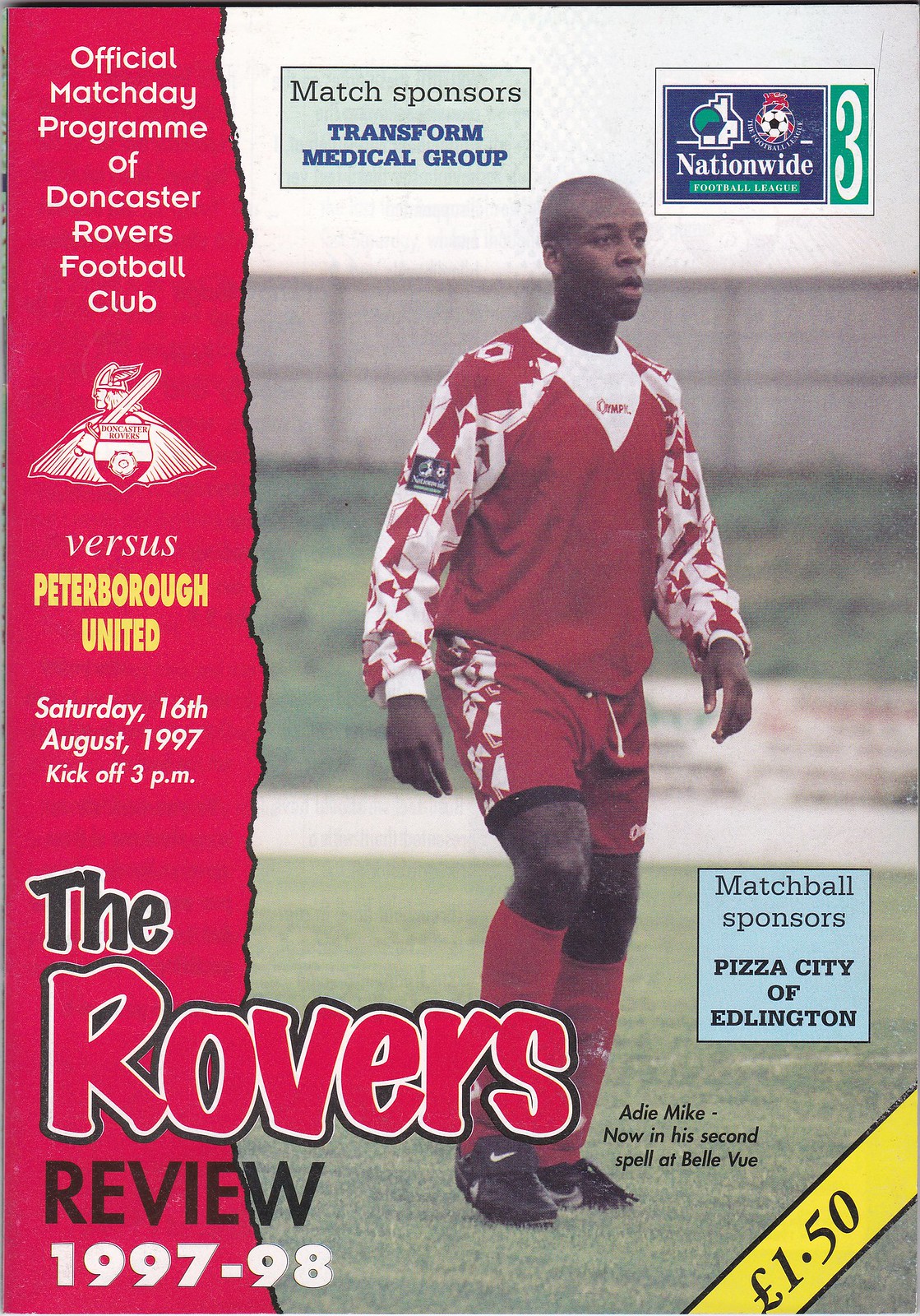The cover of the official match day program for the Doncaster Rovers Football Club features a prominent image of a soccer player, likely African-American, wearing a red jersey with white accents, red shorts with white sides, and red socks. This program is for the game against Peterborough United on Saturday, 16th August 1997, with a kickoff scheduled at 3 p.m. The top of the cover reads "Official Match Day Program of Doncaster Rovers Football Club," set against a background that transitions from top to bottom in red on the left side. In large black and red letters, the title "The Rovers Review 1997-98" stands out in the center. The top of the page also mentions "Match Sponsors: Transform Medical Group" and "Nationwide Football League." Additionally, it highlights that the match ball sponsors are Pizza City of Edlington. In the bottom right corner, the price is displayed: £1.50 against a yellow background with black text.